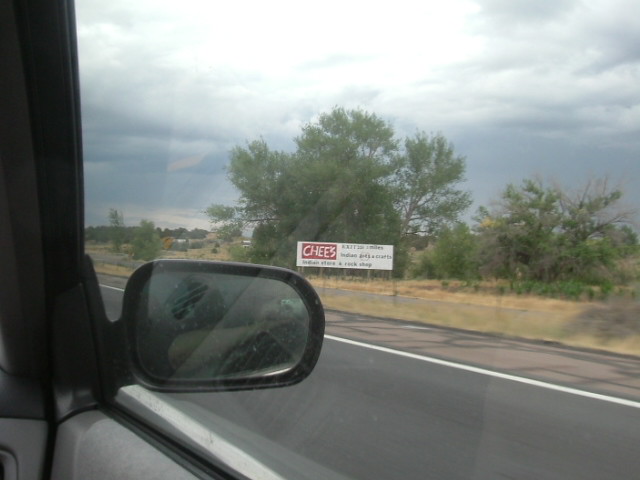A remote highway stretches ahead, its smooth black asphalt contrasting with the surrounding wilderness. A designated pull-off area is visible to the side. A large, partially obscured sign reads, "T's Best Crafted," presumably advertising a restaurant or food establishment a mile away. The backdrop is lush and green, with tall trees and open space extending into the distance. A brooding gray sky hints at an impending storm, though a single beam of sunlight pierces through a cloud, illuminating part of the scene. The image, taken from the passenger seat of a car, includes a black side mirror reflecting a person's elbow, likely the photographer.